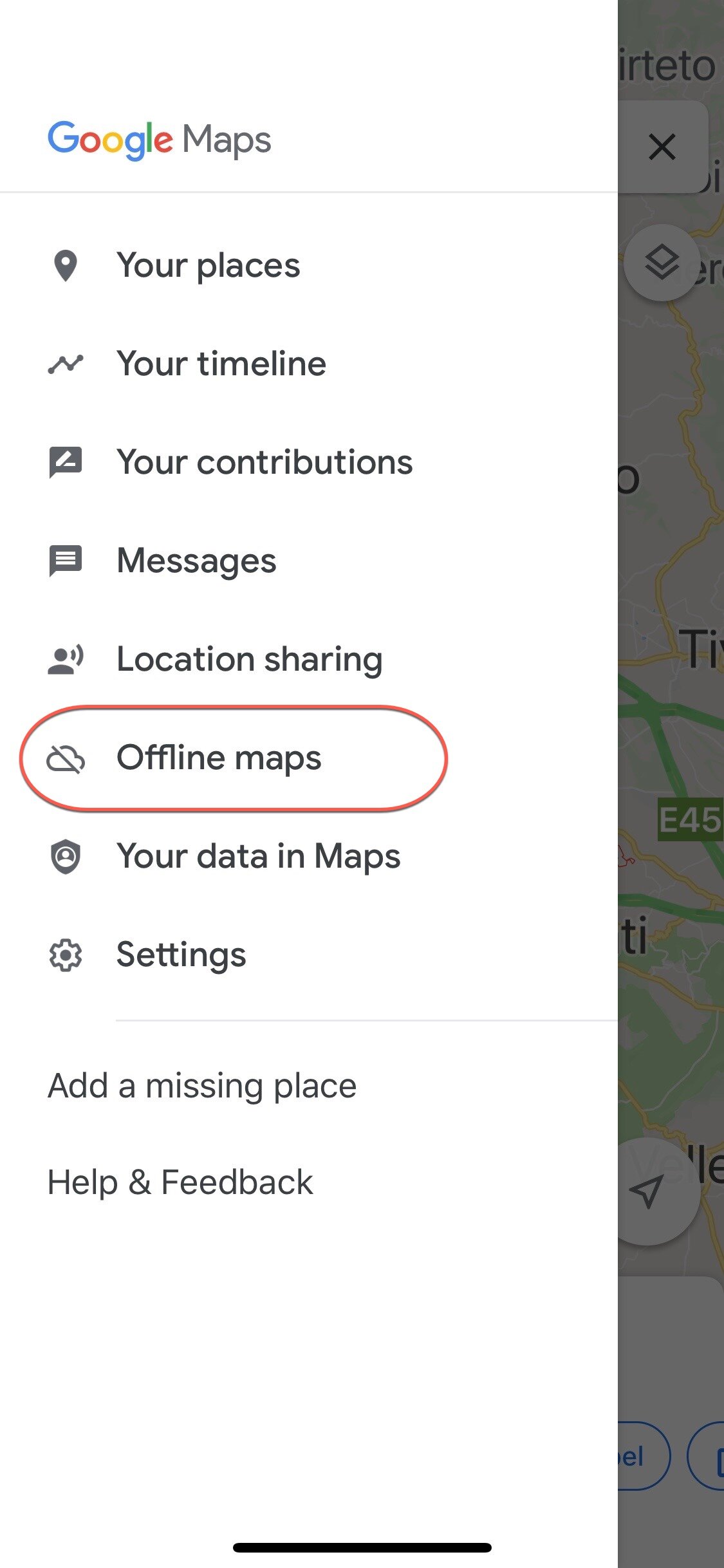A detailed screenshot of Google Maps is displayed, featuring a prominent sidebar menu. The Google Maps logo at the top left showcases the "Google" brand name in its iconic multi-colored palette of blue, red, yellow, blue, green, and red, while "Maps" is presented in a dark gray hue. Immediately below, the sidebar menu lists various options in dark gray text, including "Your places," "Your timeline," "Your contributions," "Messages," "Location sharing," and "Offline maps." This section is highlighted with a red outline, forming a rectangular shape with rounded corners. Further menu items include "Your data in Maps," "Settings," "Add a missing place," and "Help and feedback," with the last two not being bolded.

Each menu item is accompanied by a dark gray icon. Behind this sidebar, which occupies approximately 90% of the screenshot, lies the map itself, partially visible and grayed out. The map displays a network of roads and green areas denoting forests, alongside a distinct circular icon with a white background and a diagonally positioned arrow pointing to the right. The visual layering of the sidebar over the map illustrates the interactive interface of Google Maps, designed to provide users with easy access to various features and settings.